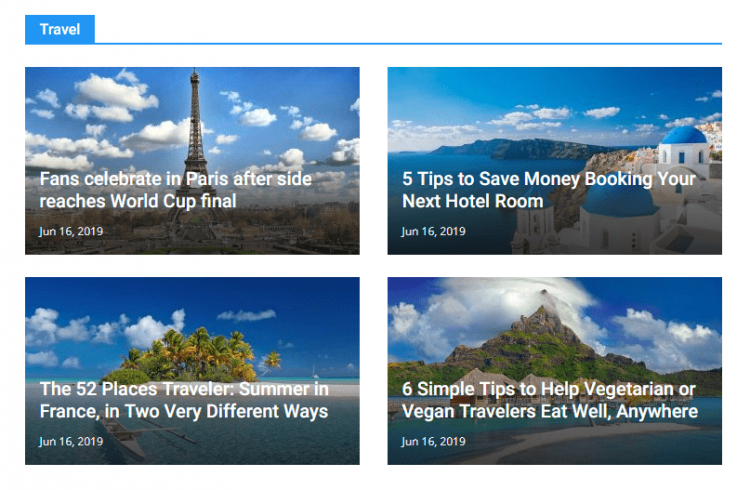The image displays a travel-themed page organized into a structured layout, with a prominent blue header section at the top, reading "Travel" in bold white letters. Below this header, a horizontal line spans the width of the page, separating the title from the content.

Beneath the line, the page is divided into four distinct sections, each featuring an image against a backdrop of clear blue skies dotted with clouds. Each section is accompanied by a title rendered in a clean, readable font.

1. **Top Left Section:** The image depicts the iconic Eiffel Tower in Paris. The accompanying title reads, "Fans Celebrate in Paris After Side Reaches World Cup Final."
2. **Top Right Section:** This image hints at a picturesque coastal city, possibly situated on a cliff. The title states, "Five Tips to Save Money Booking Your Next Hotel Room."
3. **Bottom Left Section:** Displaying a serene setting that could be either a cityscape or a countryside, this section is titled, "The 52 Places Travelers Summer in France in Two Very Different Ways."
4. **Bottom Right Section:** Featuring a tranquil, possibly beachside scene with a kayak or canoe in view, the title here reads, "Six Simple Tips to Help Vegetarian or Vegan Travelers Eat Well Anywhere."

Each section offers a glimpse into various travel destinations and helpful tips, all set against inviting blue skies infused with a sense of adventure and exploration.